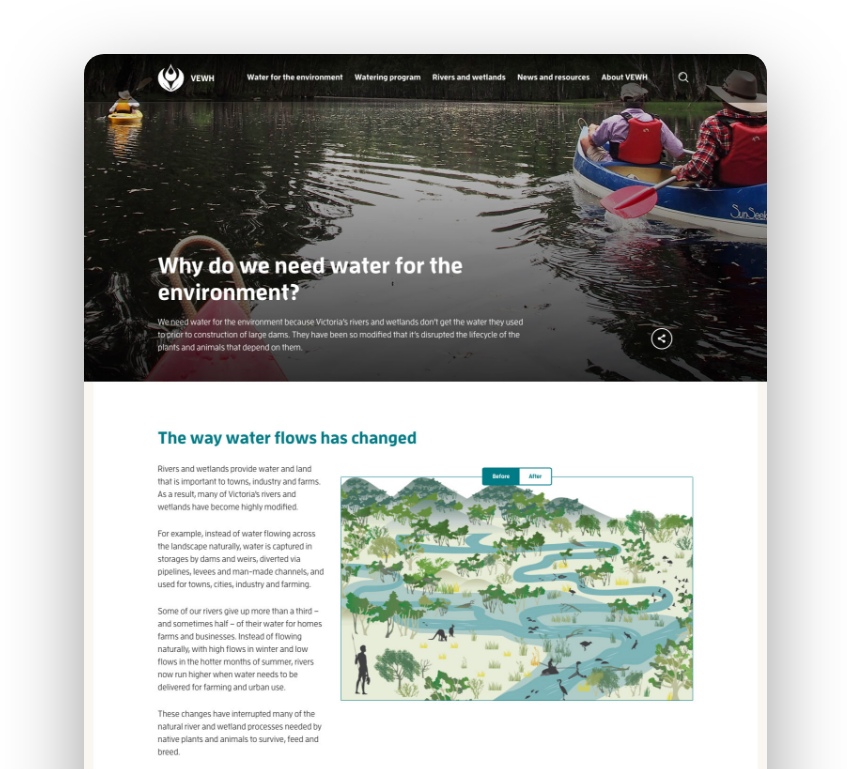In this image, we see a detailed screenshot taken from what appears to be a charity or organization’s website focusing on environmental preservation. At the top section of the website, a rhetorically engaging question is posed in bold white font: "Why do we need water for the environment?" This question is superimposed over a serene scene of two individuals paddle-boating through a tranquil body of water, emphasizing both the recreational and natural beauty of water.

Beneath this, there is an eye-catching infographic titled, "The Way Water Flows Has Changed", which presents a detailed illustration depicting prehistoric times. In the illustration, cavemen are shown interacting with a landscape where multiple bodies of water meander through a dense forest, portraying the ancient natural water systems.

Adjacent to this visual is a block of informative text discussing the historical and present changes in water flow, alongside the factors influencing these changes. The website also provides a convenient option for viewers to share this crucial information, encouraging community involvement and awareness-building. The overall composition of the screenshot effectively combines visual and textual elements to convey the importance of water in maintaining ecological balance.